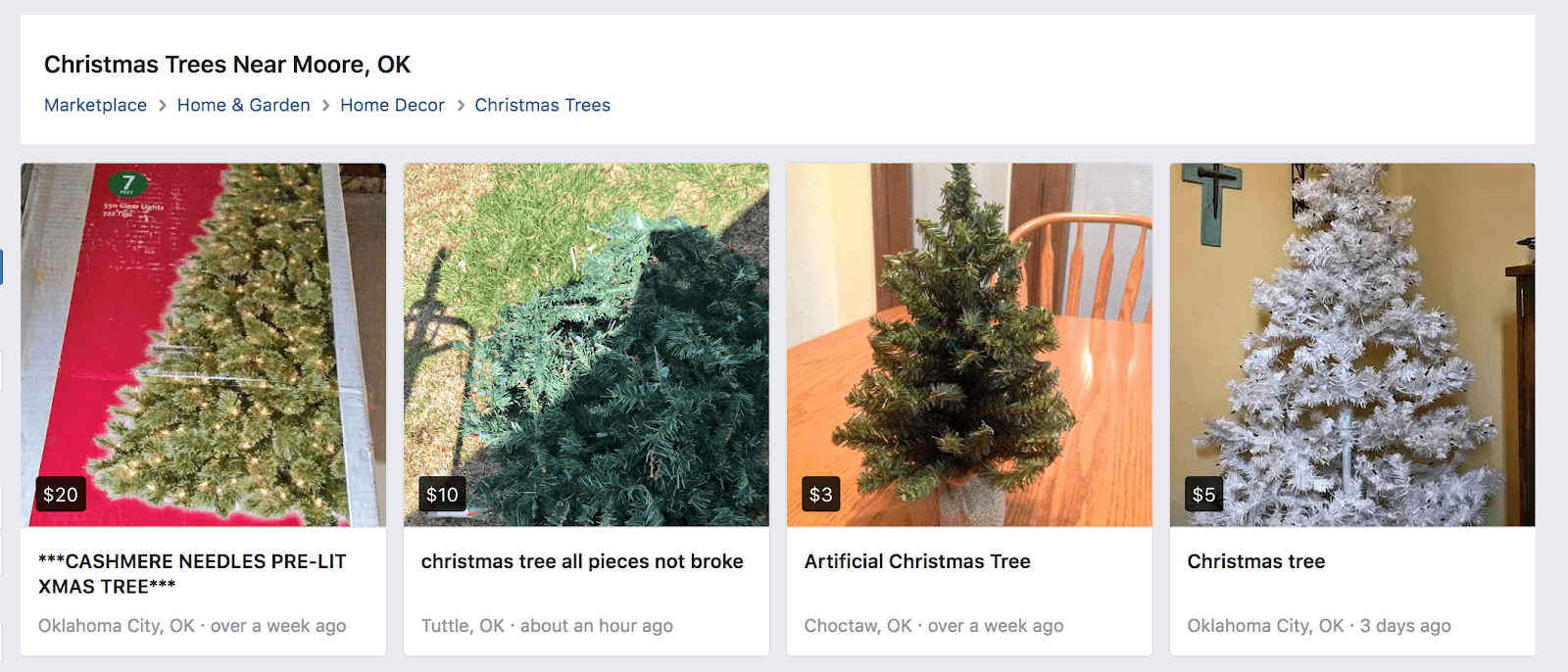A screenshot from a website showcases a section titled "Christmas trees near Moore, OK" within a white rectangle that is bordered with gray. The navigational options at the top of the page include: Marketplace, Home and Garden, Home Decor, and Christmas Trees, indicating the user's path to this display of choices.

There are four Christmas tree listings presented:

1. On the far left, a boxed, pre-lit cashmere needle Christmas tree priced at $20 is visible. The listing has three stars before and after the description. It mentions its location as Oklahoma City, OK, and was posted over a week ago.

2. Next to it, a $10 tree is partially shaded and lying on grass. The description reads: "Christmas Tree, All Pieces, Not Broken," and it is in Tuttle, Oklahoma. This listing was added about an hour ago.

3. To the right, there is a very small tabletop tree priced at $3, described as an "Artificial Christmas Tree." Its location is Choctaw, Oklahoma, and it was listed over a week ago.

4. The last listing on the far right shows a white Christmas tree inside a house, priced at $5. This tree is located in Oklahoma City, OK, and was posted three days ago.

Each listing provides brief details about the product, its condition, location, and the time since it was posted.